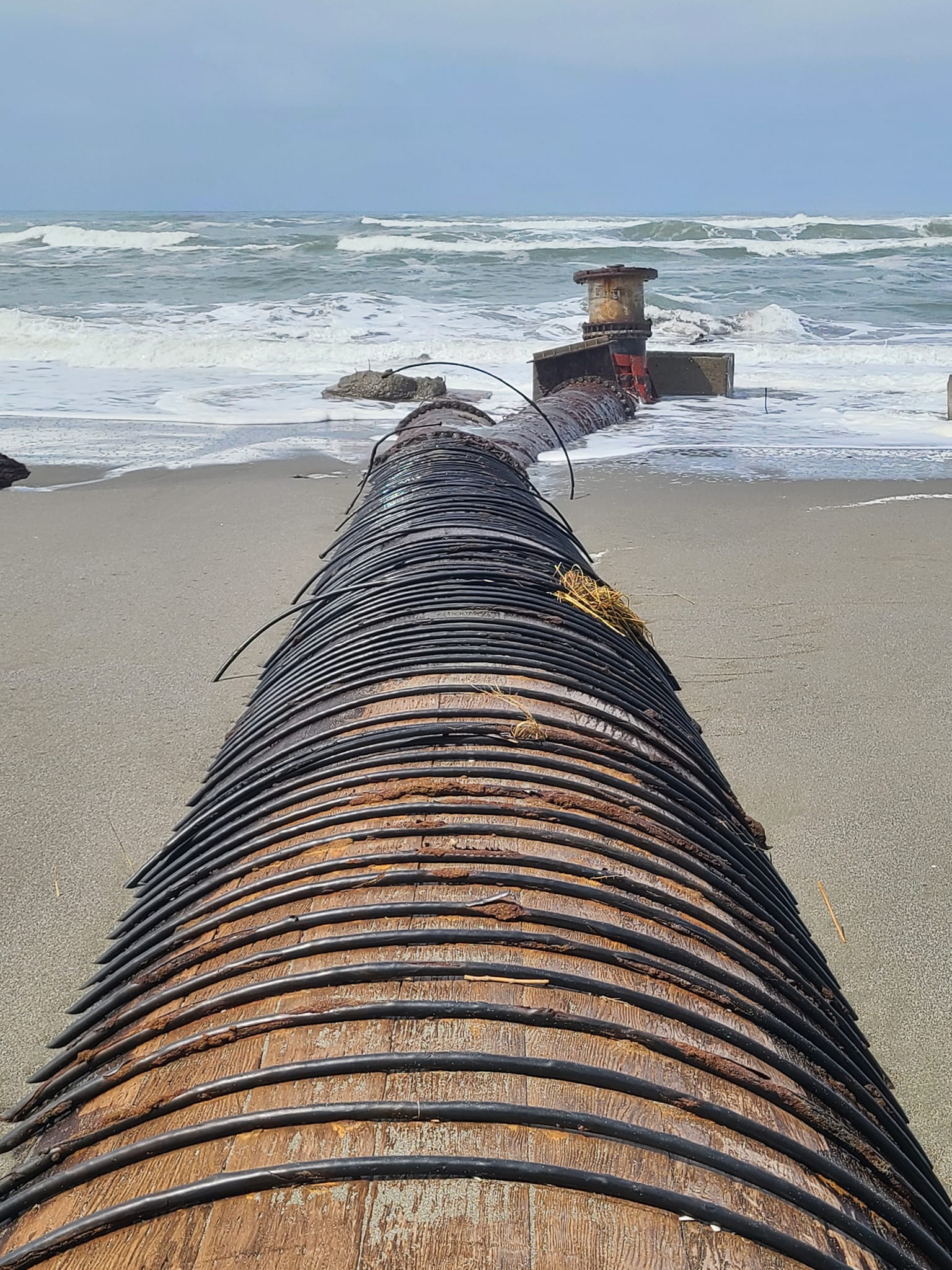This is a detailed beachside scene captured in a photograph during the daytime. Dominating the middle of the image is a large cylindrical pipe, constructed from wooden planks aligned lengthwise and secured by closely spaced, thick steel or metal bands. The pipe extends from the sandy beach, where the sand is a darker grayish brown color, all the way into the rough, greenish-blue waves with white caps and sea foam. As the pipe reaches the ocean, it transitions into a vertical cylinder with a broader top, accompanied by concrete structures around it, including a tipped-over cinder block. To the left of this, there is a pile of large rocks or possibly cylindrical cinder blocks. The sky above is a cyan hue with hints of white, emphasizing the daytime setting. Something red is also present near the crashing waves in the background.